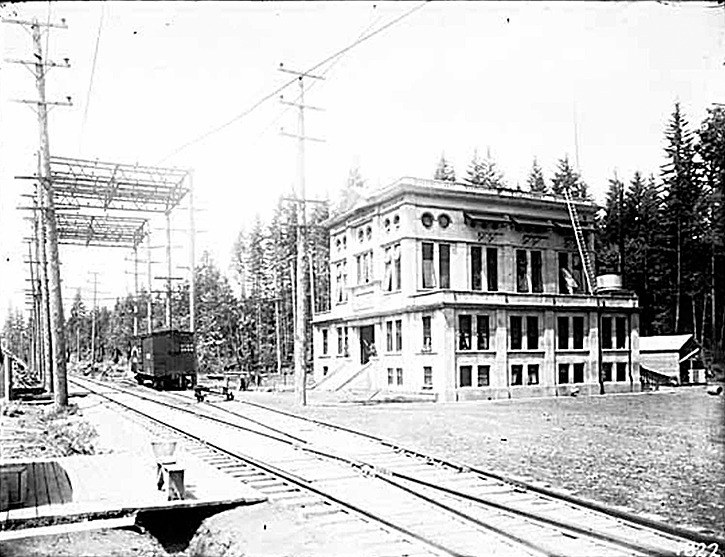This appears to be a historical black and white photograph depicting a railroad scene, possibly from 1922, despite the date "1822" inscribed at the bottom, which predates the advent of photography. The image features two parallel railroad tracks that start at the bottom right corner, extending towards the center-left of the frame, crossing over early on. Above and around the tracks are numerous trestles and electrical poles, with some forming a square-like shape overhead. 

In the background, there's a prominent two or three-story stone building, likely a train station or a courthouse, characterized by its large, white marble appearance and tall windows with shutters on the upper stories. The building has a wide set of stairs leading to the main entrance, and a ladder is visible going up to the roof. Behind this building stands a cluster of large pine trees and a small shed.

On the right side of the tracks sits a vintage car, while the left side appears open. In the foreground, a wooden plank bridges a ditch adjacent to the rail line, adding to the aged and industrial ambiance of the scene.